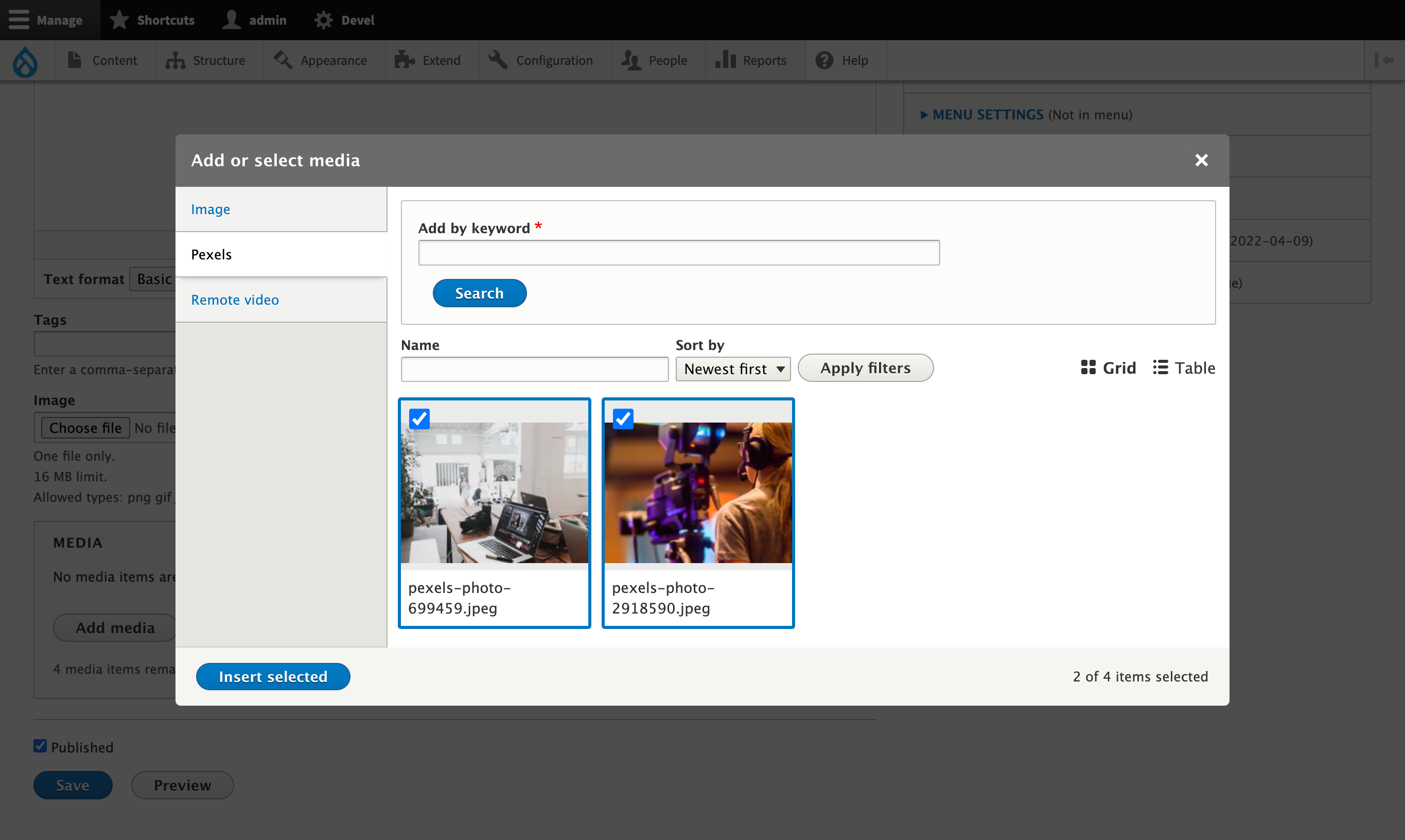An urgent scene unfolds in the background, showcasing the complex management of multiple administrative tasks. This intricate environment features a range of options such as shortcuts, administrative controls, content development, and structural organization. The interface is packed with tabs for appearance customization, extension integration, configuration settings, user management, report generation, and help support.

An image selection interface prominently displays various media options, including the ability to add or select media files. Users can choose from images or remote videos, add media by keyword, or search by name. Advanced options allow for sorting by newest first, applying filters, and viewing items in a grid or table format. Among the selected sources are images labeled as pixelsphoto699459.jpg and pixels-photo2918590.jpg, highlighting the meticulous selection process tailored to the current needs.